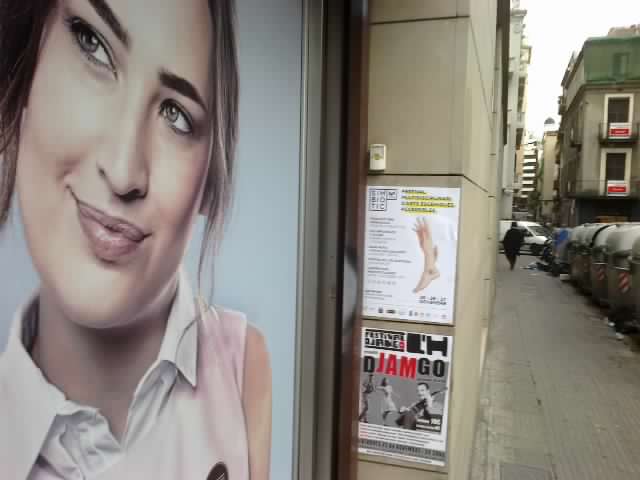The image captures a scene taken from the end of a sidewalk, looking down a street to the right. A significant portion of the view is bisected by a stone building wall, which features a sensor and two posters—one possibly advertising physiotherapy and the other an event. To the left, a large window of a storefront—perhaps a hair salon—dominates with an advertisement. This poster features a cartoonish depiction of a woman with dark eyebrows and brown hair, tied back but unseen, wearing a sleeveless white collared shirt and set against a blue background. She is pursing her lips and looking to her right. The right side of the wall reveals a long sidewalk lined with several parked cars. At the far end of the sidewalk, a white van is seen emerging from a perpendicular street while a person in a winter coat walks towards it.